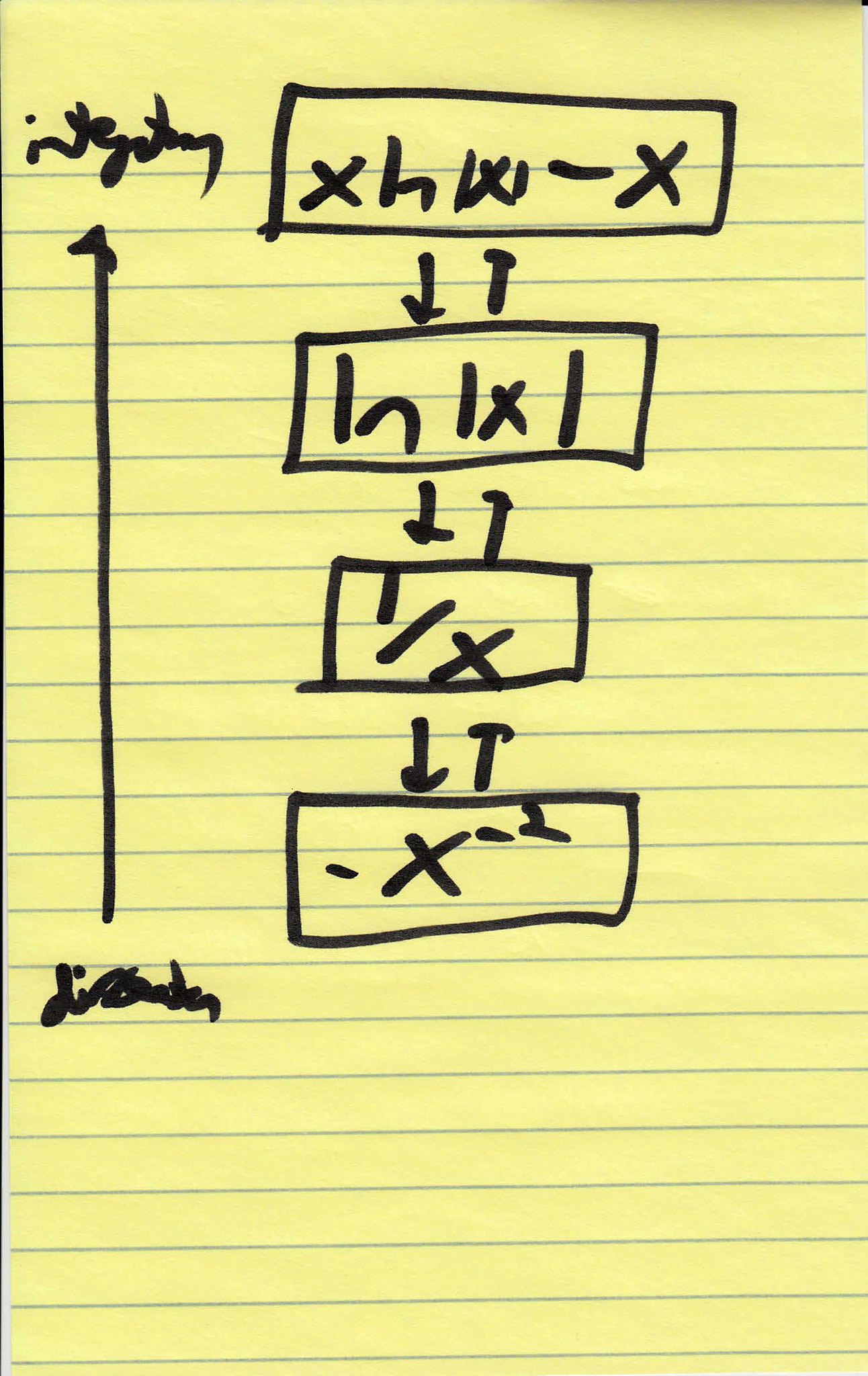The image features a piece of yellowish lined paper with blue horizontal lines. On the left side of the paper, there's a long vertical line ending in an arrow at the tip. At the top of this arrow is an inscription, seemingly "I-N-T-G-A-T-I-Y," though it is not entirely clear.

At the bottom of the arrow, the word "DISORDER" is written prominently. The text across the paper appears to be written using a black marker pen. 

On the right side of the paper, adjacent to the arrow, there is a long horizontal rectangle near the top. Inside this rectangle are the characters "X-H-1-X-1-X." Below this, another arrow points downward. Close to this arrow is a "T" on its side. Further down, there is another horizontal rectangle containing the text "1-N-1-X-1." 

The paper also features two additional arrows, one pointing downwards and the other upwards, coupled with a smaller rectangle at the bottom containing the fraction "1/X." The arrows continue with the downward arrow positioned on the left and the upward arrow on the right. Finally, there is a longer arrow with the notations "-X" and "-X²" at the top right.

The entire sketch appears to depict some form of structured data or a schematic diagram with various annotations and mathematical notations.